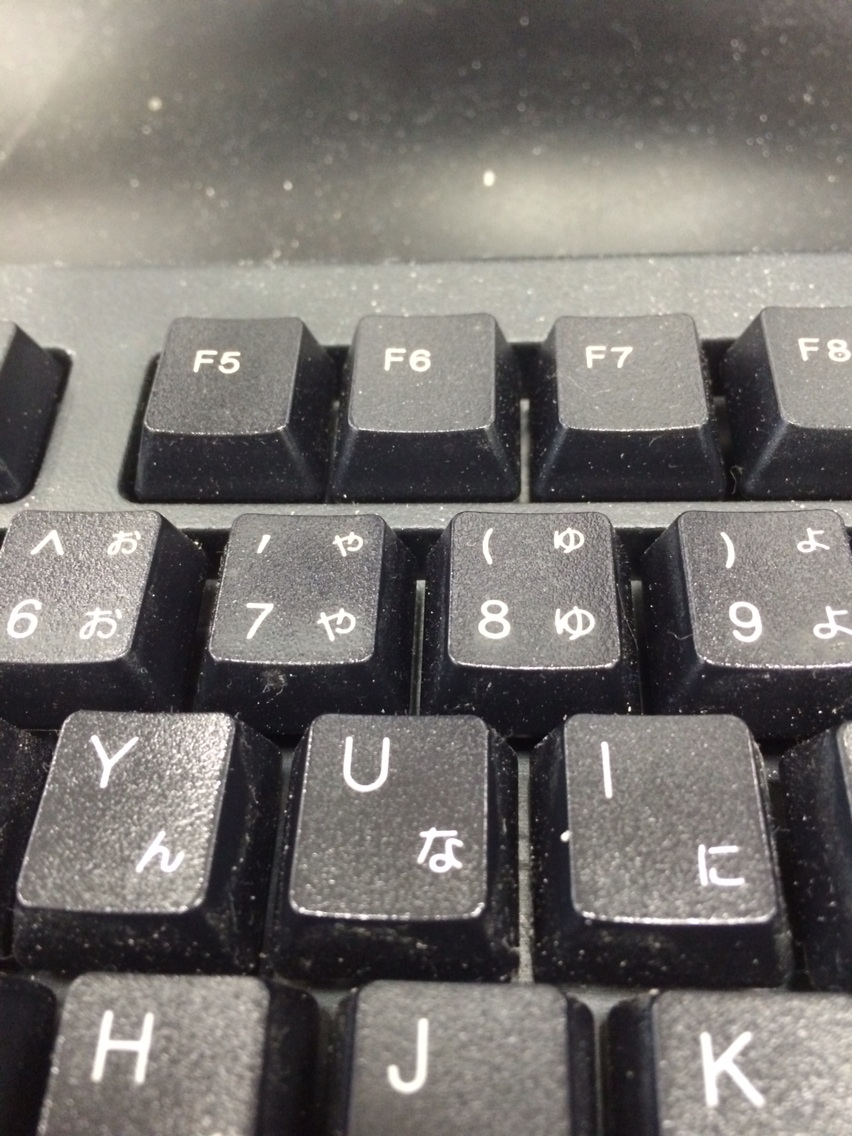This close-up photograph captures a detailed portion of a black computer keyboard. The keys feature white Latin letters and alternate characters, suspected to be Japanese, displayed in the bottom right corner. The visible key rows include the top row with F5, F6, F7, and F8, followed by the numbers 6, 7, 8, and 9 in the next row. Below these, the letters Y, U, and I are showcased, and the row beneath features H, J, and K. The keyboard surface is noticeably dirty, with specks of dust scattered across the keys. A strong overhead light source creates a glare, slightly overexposing some keys. The photograph predominantly uses gray, white, and black tones, with the background at the top appearing as an out-of-focus blur in gray.